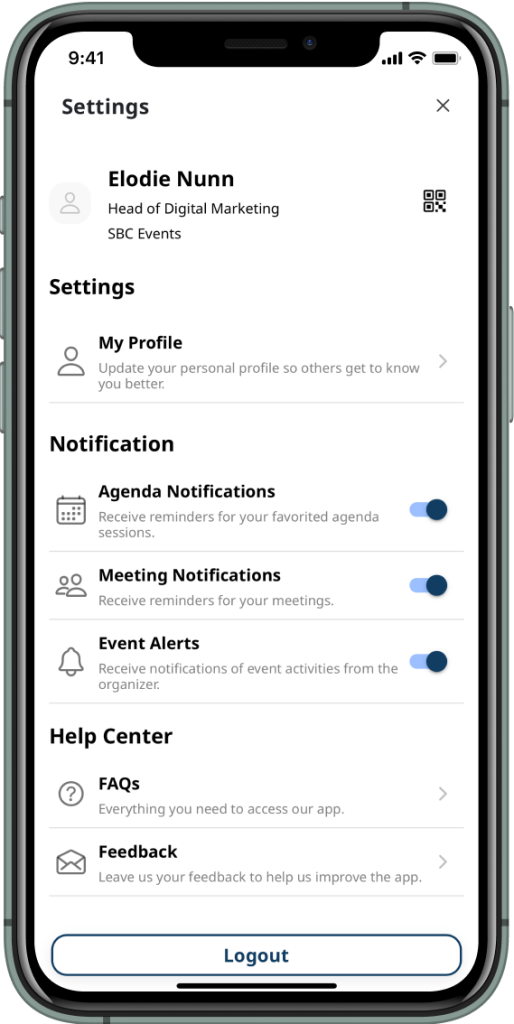This detailed caption describes a digital mock-up of a company's app interface on a smartphone. The image features a mostly white background with various UI elements presented.

At the top of the interface, the left-hand side displays the time "9:41" without indicating AM or PM. On the right-hand side, icons indicate full cell signal, full Wi-Fi signal, and a fully charged battery.

Below this information, there is a bold black heading reading "Settings." This section displays a user profile that includes a silhouette icon of a person composed of a half-crescent moon within a circle. The profile name "Elodie Nunn" is written below the icon, followed by the title "Head of Digital Marketing" and "SBC Events."

On the right side of the profile, there is a QR code featuring three distinct squares. Below this, another bold black heading reads "My Profile," accompanied by an icon of a person with a turned-over half-crescent moon representing the head. Below this, in gray text, is an invitation to "Update your personal profile so others get to know you better," followed by a right-pointing arrow.

The next section features a calendar icon labeled "Agenda Notifications," with gray text underneath stating "Receive reminders for your favorite agenda sessions" and a blue, selected slider. Similarly, another option with a blue, selected slider reads "Meeting Notifications," presented with an icon of two people and the description "Receive reminders for your meetings."

Following this, there is an "Event Alerts" option marked by a bell icon. Finally, a bold heading titled "Help Center" includes a circle with a question mark and another bold heading "FAQs" with the description "Everything you need to access our app" in non-bold text.

Further down, there is an icon of an open envelope labeled "Feedback" in bold black, inviting users to "Leave us your feedback and we'll be happy to answer any questions." This is paired with a question mark icon and bold "FAQs" with the text "Leave us your feedback to help us improve the app," both accompanied by arrows.

At the bottom of the interface, there is a blue oval button with blue text in the center reading "Log Out."